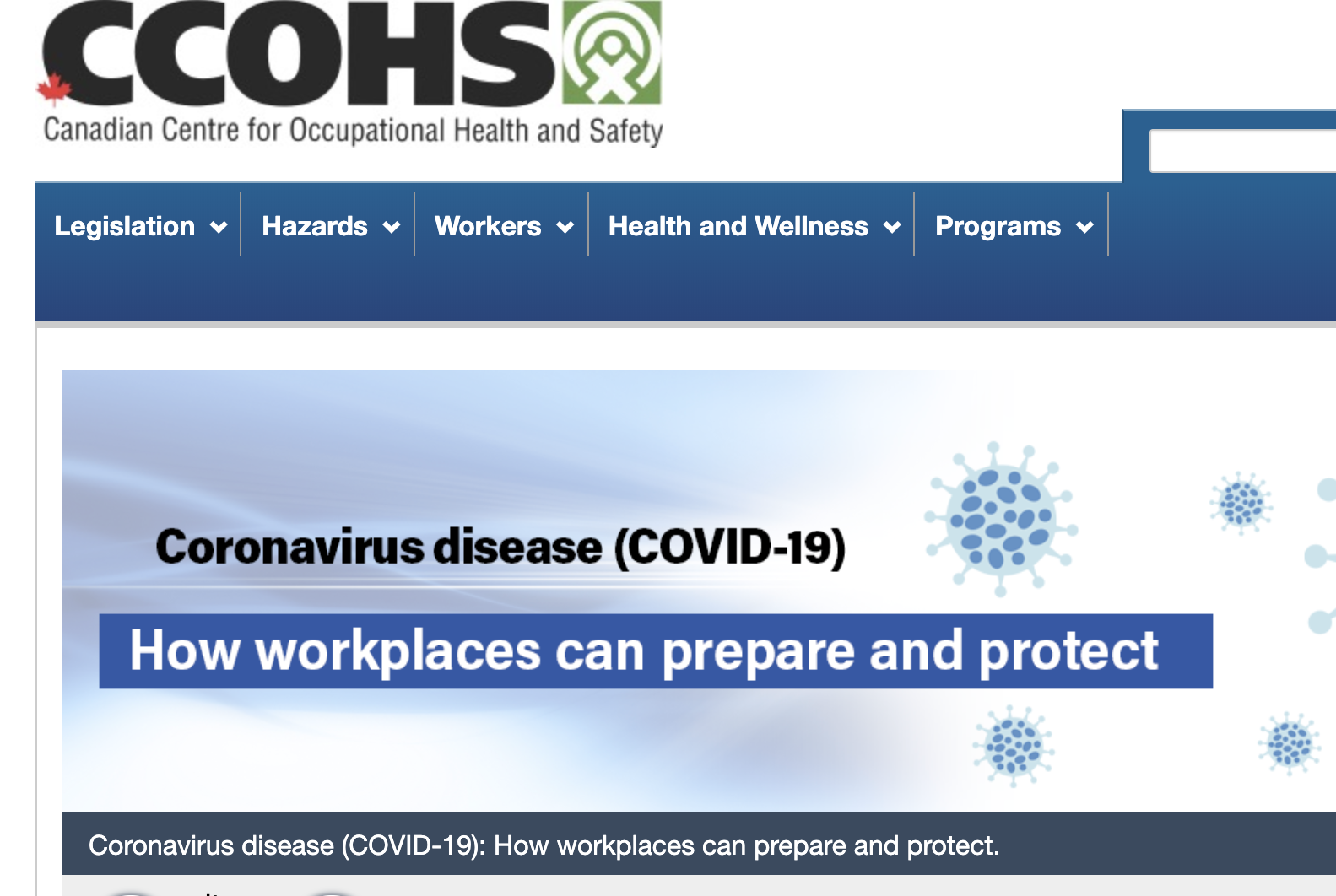The Canadian Centre for Occupational Health and Safety (CCOHS) Website

The top left corner of this website features the CCOHS logo: a green square with a white circle in the center, containing a symbol that resembles an 'X' or a stick figure. Adjacent to the first 'C' in the logo is a small red maple leaf, highlighting its Canadian origin. Below the logo, there is a prominent blue navigation bar that includes drop-down menus for various categories like Hazards, Workers, and Health and Wellness Programs.

The main body of the website predominantly uses shades of blue and includes key information in black font, stating "Coronavirus Disease, COVID-19." Directly below this, in white lettering, is the message: "How Workplaces Can Prepare and Protect." The site also features illustrations of the coronavirus, adding a visual element to the information provided.